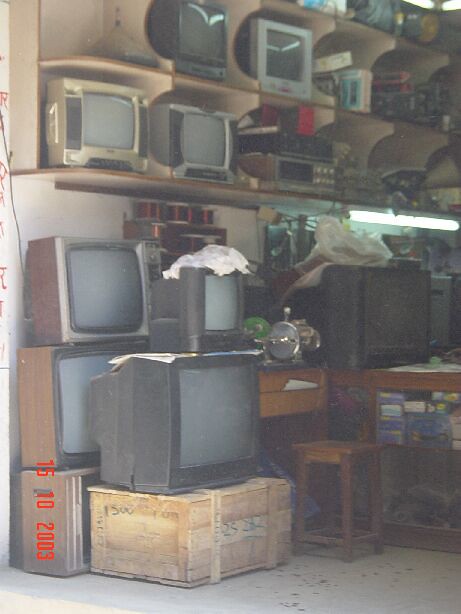This slightly blurry photograph, taken on October 15, 2003, according to the red date stamp in the bottom left corner, depicts the cluttered interior of what appears to be a storage unit, old electronics store, or television repair shop. The area is filled with an assortment of retro CRT televisions, VCRs, and videotapes. The TVs come in a variety of sizes and colors, ranging from small, kitchen-sized sets to larger, bulkier models. These TVs are either stacked on the floor or placed on wooden shelves lining the walls, with some sitting atop crates and makeshift wooden furniture. The smaller sets are organized within cubby holes, while others are precariously balanced on top of each other. A wooden stool and a fluorescent light can also be seen amidst the dusty and disorganized space. The concrete floor is marked by a white surface with black spots, adding to the overall messy and sloppy appearance of the room.